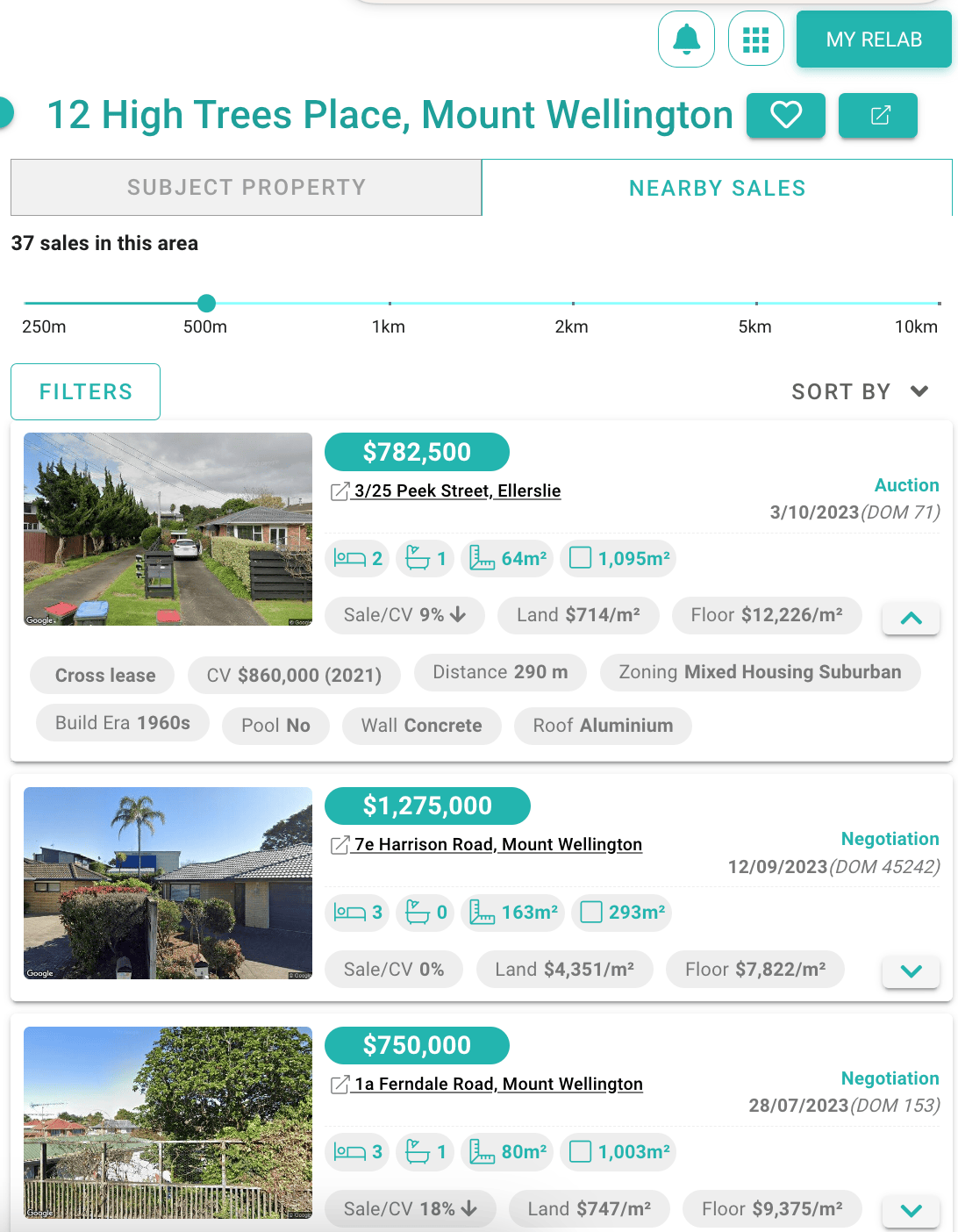Screenshot of a real estate listing featuring multiple properties for sale or rent in the Mount Wellington area. At the top, the listing header reads "12 Hightree Place, Mount Wellington" with a note mentioning "37 sales in the area."

1. **Property:** 325 Peak Street, Ellerslie
   - **Price:** $782,500
   - **Details:** 2 bedrooms, 1 bathroom
   - **Area:** 64 square meters (interior), 1,095 square meters (land)

2. **Property:** 70 Harrison Road, Mount Wellington
   - **Price:** $1,275,000
   - **Details:** 3 bedrooms, no bathrooms listed
   - **Area:** 163 square meters (interior), 293 square meters (land)

3. **Property:** 1A Ferndale Road, Mount Wellington
   - **Price:** $750,000
   - **Details:** 3 bedrooms, 1 bathroom

The listing presents a snapshot of real estate options, highlighting key features such as price, bedroom and bathroom count, and property dimensions.